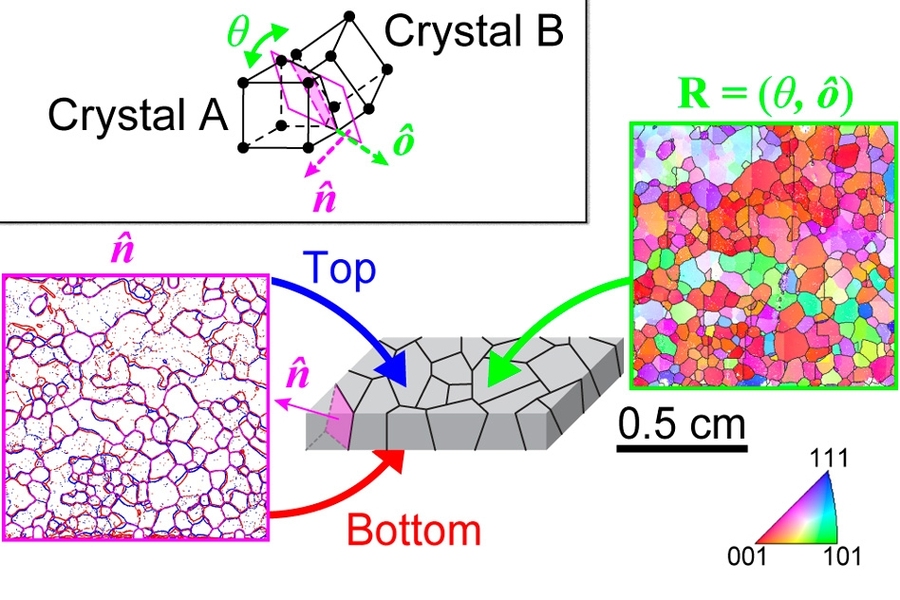This diagram features a detailed illustration on a white background, primarily showcasing relationships between crystalline structures and patterns. On the top left, there's a black geometrical shape labeled "crystal A" and "crystal B," connected by black lines and dots. Below this, a purple square contains irregular purple wiggly lines with two arrows emerging from it—a blue arrow pointing right and down, and a red arrow pointing right and up. Both arrows terminate at a green cuboidal structure on the right side of the image.

On the far right, there's a green square filled with multicolored patterns, annotated with the formula "R = 0,0" and a measurement of "0.5 cm." An additional green arrow from this square also points toward the green cuboid in the center. At the bottom right, a colorful triangle is marked with labels "111," "101," and "001." The diagram includes annotations and varied color coding to highlight different scientific concepts and data, likely related to crystal structures and their lattice patterns.